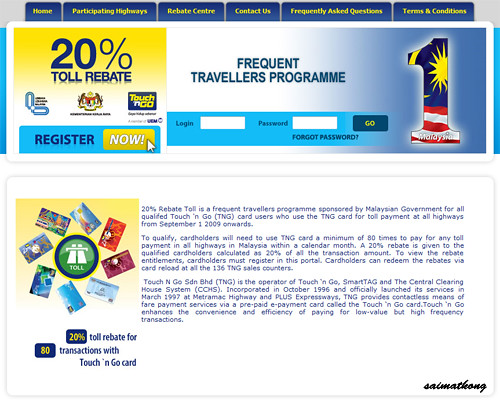This image depicts a promotional web page for the "Frequent Travelers Program," a 20% toll rebate initiative offered to frequent highway users in Malaysia. The page header features navigation options including "Home," "Participating Highways," "Rebate Center," "Contact Us," "Frequently Asked Questions," and "Terms and Conditions." Prominently displayed is the announcement of a 20% toll rebate for users who complete 80 transactions using Touch 'n Go cards in a calendar month. 

Below the informative text, a visually appealing graphic shows a series of Touch 'n Go cards encircling a blue circle with a green center and a white symbol labeled "Toll." Adjacent to this, text elaborates that the 20% rebate is part of a program sponsored by the Malaysian government to reward frequent users. It specifies that users qualify by making a minimum of 80 toll payments on highways in Malaysia within a month, with the rebate amount being 20% of the transaction total.

The page also includes sections for users to "Register Now" and "Log In," with white text fields for username and password and a "Forgot Password" link beneath. An American flag with the number 1 is displayed to symbolize high standards or leadership. The bottom of the image notes that the program is operated by the firm that manages the Touch 'n Go Smart Tag system, initially incorporated in October 1996 and officially launched in 1997 at Metramac Highway and PLUS Expressways. This initiative aims to enhance the convenience and efficiency of handling low-value, high-frequency toll transactions.